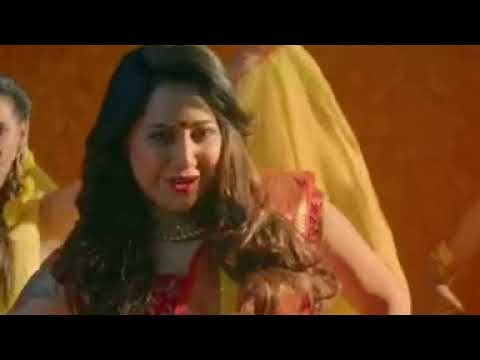In this high-definition image, a still shot that seems like it’s from a Bollywood film, a striking Indian woman is captured mid-dance. She stands in a dynamic pose, adorned in a vibrant, elaborate red sari accented with yellow and gold details. A conspicuous red bindi adorns her forehead, complementing her pink lips and dark, flowing hair. Around her neck, a thick, golden necklace sparkles under the sunlight which illuminates the left side of her face, suggesting the scene is outdoors. Flanking her in the background, two other dancers, also elaborately dressed in yellow and white drapery that might be saris, serve as subtle, supporting figures. The backdrop is a fiery red, shading into a rusty brown hue, creating a dramatic contrast with the performers' attire. The image radiates energy and cultural vibrance as the woman appears to be either dancing, performing, or possibly even singing, caught in an expressive moment that feels very much like a captivating frame from a Bollywood dance number.